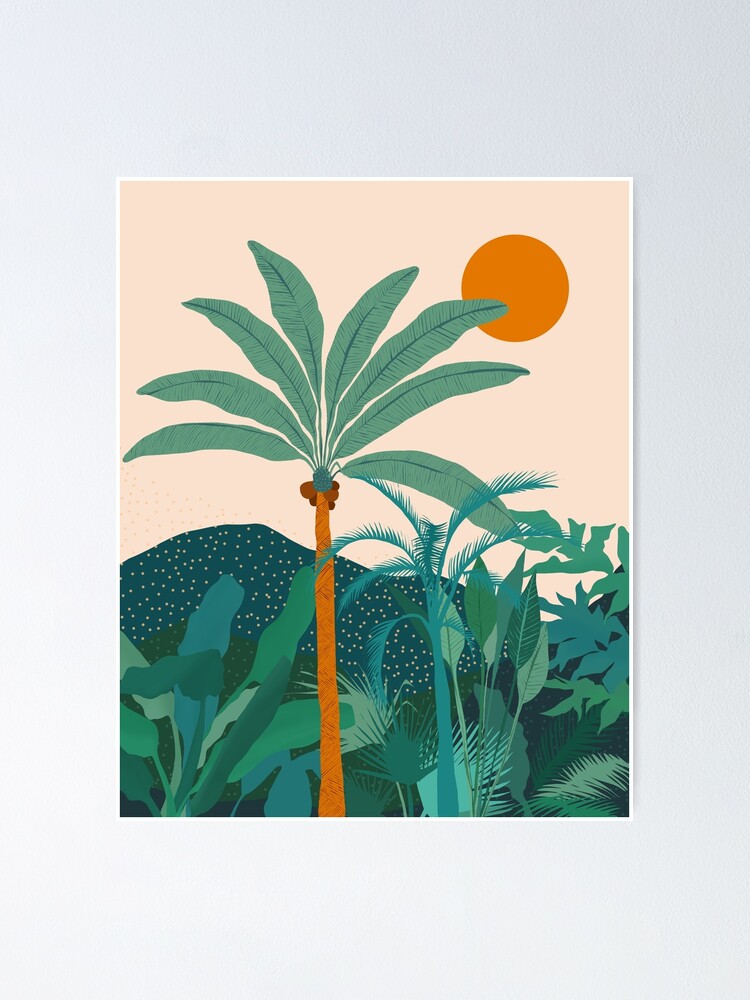The image depicts a piece of artwork hanging on a neutral light blue wall with a thin white border. The artwork illustrates a minimalistic forest scene, characterized by numerous types of trees and plants in various shades of green, depicted primarily through their contours with minimal internal details. Prominently featured in the center is a coconut palm tree with a distinctive orange trunk, large green fronds, and brown coconuts beneath its leaves. In the background, a dark green mountain range adorned with small yellow dots stretches across the scene, while a salmon-pink sky provides an ethereal backdrop. An orange sun, perfectly circular, is positioned in the upper right corner of the painting, adding warmth to the tranquil landscape.